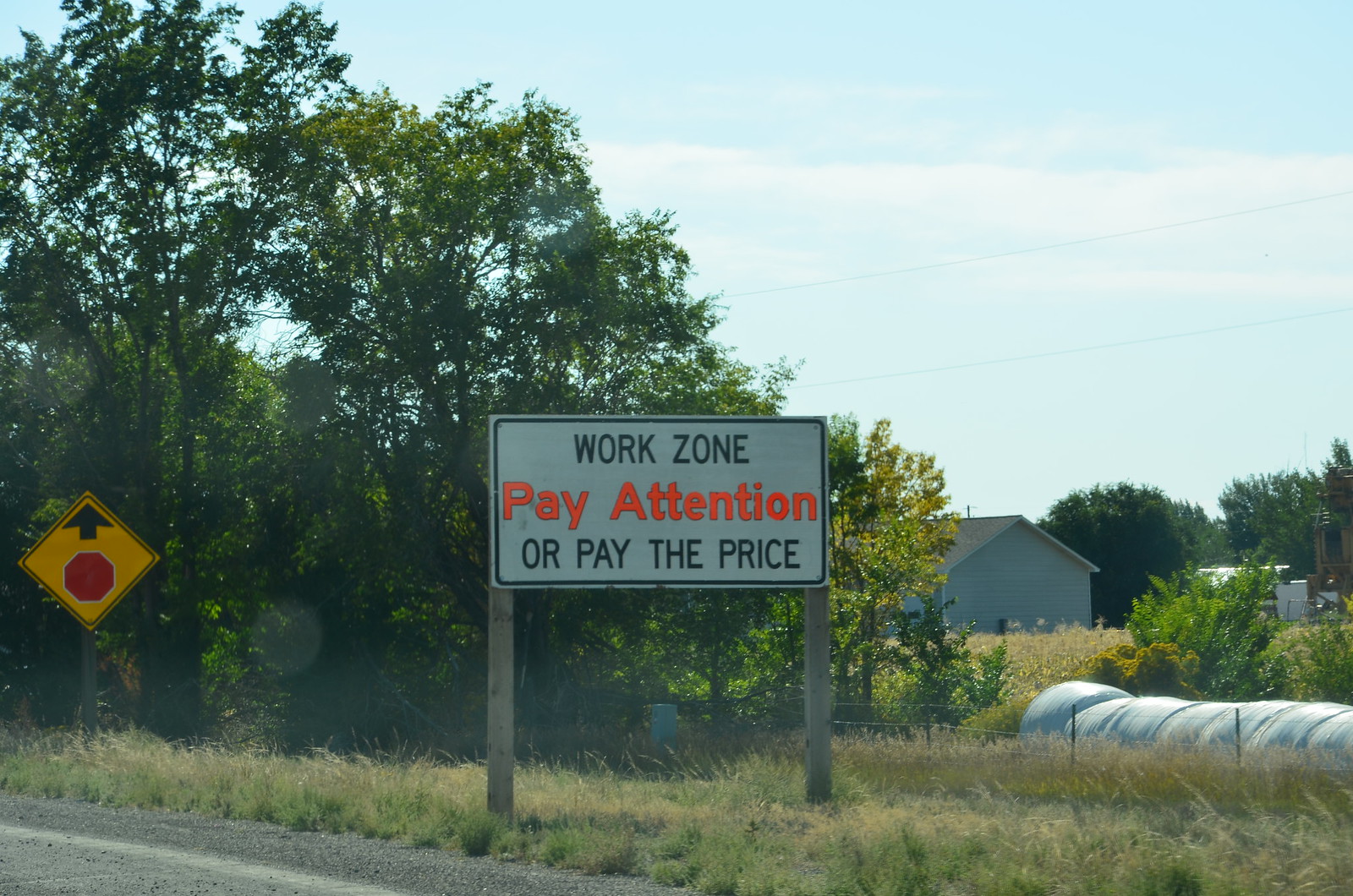The image is set outdoors showcasing an expansive scene underneath a light blue sky accented by white clouds. In the background, there is a house or building with a sloped brown roof, to the right of which stands a cluster of darker green trees. The foreground presents a mixture of landscapes including grasslands, lower-level bushes, and a patch of gravel. To the left, a slender farmer's fence and a white plastic-wrapped hay bale are visible. The right side of the image features a highway marked by a white line.

Prominently displayed in the scene is a large white road sign with a black border standing secured to two wooden posts. The sign reads "Work Zone" at the top in black letters, beneath which "Pay Attention" is written in bright orange, followed by "Or Pay the Price" in black. Directly behind this main sign, slightly to the right, is a yellow diamond-shaped traffic sign with a black arrow and the silhouette of a stop sign, indicating a stop sign ahead.

Additional elements include tall grass with brown weeds in the middle ground and a small concrete patch seen near the bottom left corner. Overall, the image captures a tranquil roadside scene marked by clear safety signage against the backdrop of varied vegetation and rural elements.